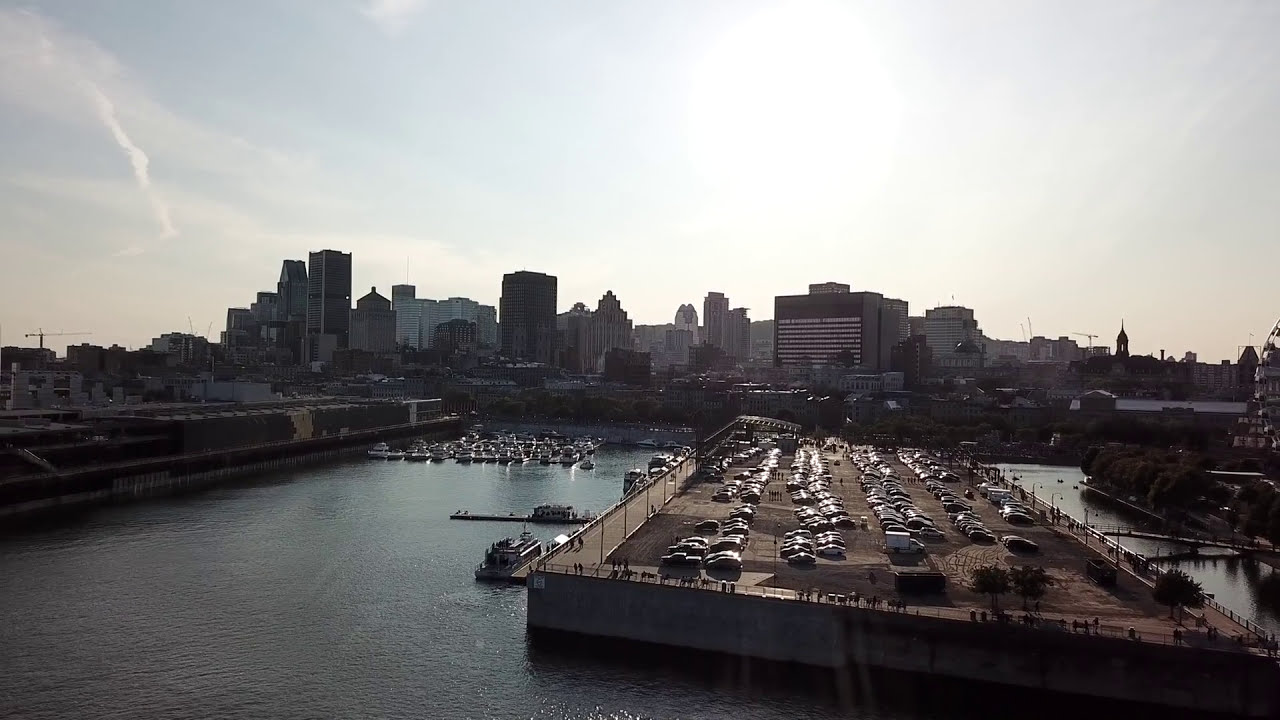This photograph showcases a bustling cityscape on a bright, sunny day with wispy clouds creating a hazy atmosphere. The foreground features a wide concrete dock, jutting out into the harbor, serving as a large parking lot filled with approximately a hundred cars and a few small trucks. People can be seen walking along a roadway that borders the dock. To the left side of the image, several boats are moored closely to the city’s skyline which is composed of moderate-height buildings and visible construction cranes. A slender bridge extends from the dock towards the right. In the background, beyond the harbor’s U-shaped water, is an array of taller skyscrapers, with the sun either rising or setting behind them, casting a warm glare through the hazy clouds.